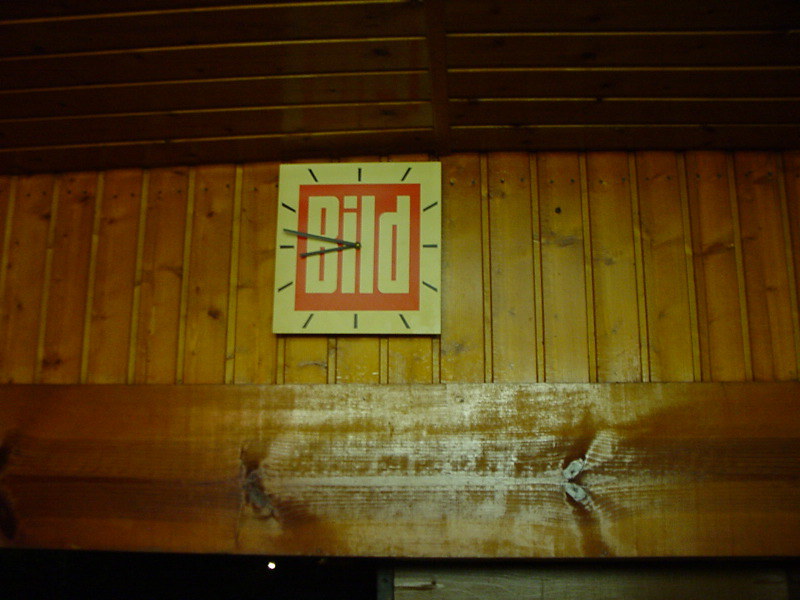The photograph presents a meticulously detailed view of a wood-paneled wall, captured in landscape orientation. The dominating presence of pine wood, with its natural finish, creates a warm and rustic atmosphere. The upper part of the image showcases horizontal wooden planks, suggesting they might serve as the ceiling, seamlessly matching the paneling on the wall. Just below this ceiling area, a short segment of wall extends, topped by a robust plank approximately 10 to 12 inches in width that stretches across the frame from left to right. This prominent board is rich with natural details, including visible knots and wood grain, catching a faint glare of light near its center.

In the lower section of the image, a narrow strip reveals contrasting elements: a black area with a small white dot of light on the left, and an ambiguous surface on the right that might be a wall or concrete, adding a mysterious touch to the composition.

Mounted on this pine-paneled wall is a distinctive square clock. The clock, presumably battery-operated due to the absence of any visible wiring, features a stark white body with a striking red square at its center. The red square prominently displays the word "BUILD" in bold white letters. The clock face lacks numerical markers, instead opting for black lines to indicate each hour. Notably absent is a second hand, leaving only the hour and minute hands, which point to approximately 13 minutes before 9 o'clock. The overall scene is a harmonious blend of natural wood textures and minimalist timekeeping design.